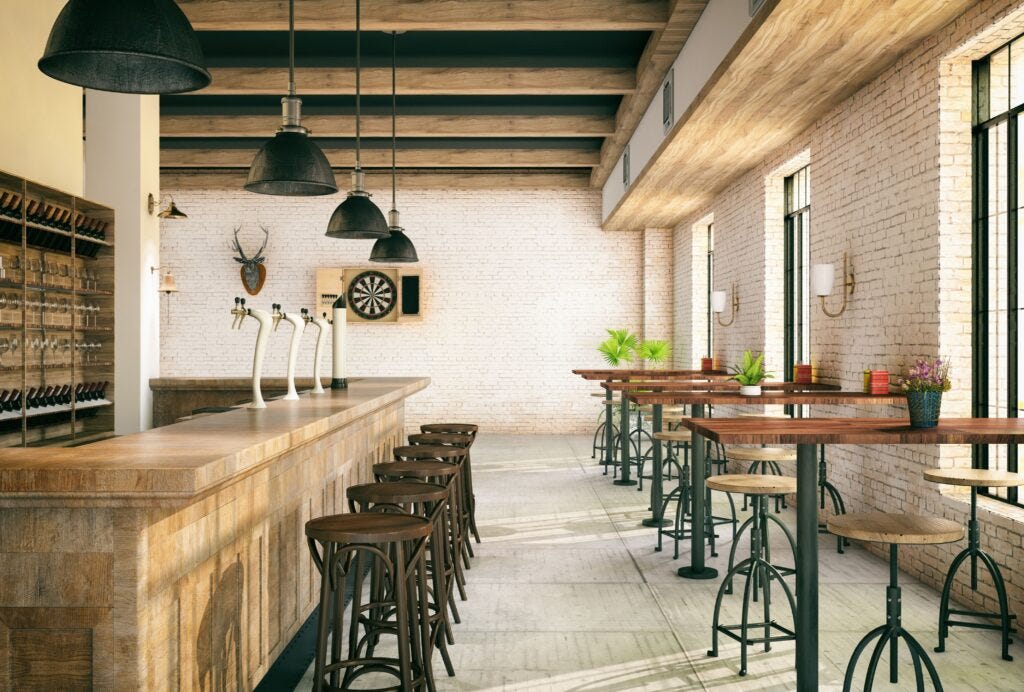This is a detailed photograph of the interior of a modern, clean restaurant featuring a spacious bar area and seating. On the left-hand side, there's a wine bar with a light wooden bar top running its length. This bar area is decorated with industrial-style elements including three beer tap spouts and black metal light shades hanging low from the wooden ceiling beams. Adjacent to the bar, there’s a prominent wine cabinet wall that neatly holds a variety of wine bottles and glasses. In front of the bar, five dark, industrial-looking bar stools with dark wood seats are neatly arranged.

On the right-hand side of the image, the room features four high-top tables with dark brown, shiny wooden tops. Each table is supported by a black cylinder base and is paired with high bar stools with black metal bodies and light teak wooden seats. The right-hand wall is constructed from white brick and houses several potted plants and red boxes placed on the table tops, creating a warm atmosphere. Sunlight pours in through three large windows on this wall, illuminating the space. Additionally, white light fixtures are affixed between the windows, enhancing the modern aesthetic.

The back wall of the restaurant, also sporting white brick, hosts a mounted deer head and a dartboard—adding a rustic charm to the venue. Above this area, more black lights hang from the ceiling, matching those above the bar. The wooden roof with its long beams ties the whole area together, highlighting the cohesive blend of modern and rustic features throughout the restaurant.